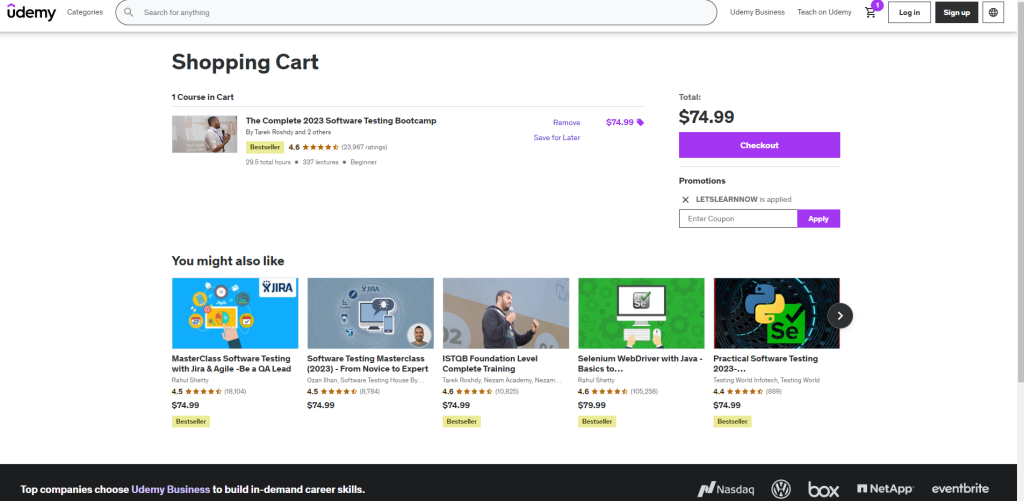At the top of the image, a white rectangle features the Udemy logo on the left. To the right of the logo, there is a "Search for anything" bar, followed by a "Log In" button, a "Sign Up" button, and a shopping cart icon labeled "Shopping Cart." The cart currently holds one course: "The Complete 2020 Software Testing Bootcamp," priced at $74.99, displayed to the left of a bold purple "Checkout" button.

Below the checkout section, a recommendation section titled "You may also like" presents five courses in rectangles, each with a corresponding image:

1. "Masterclass Software Testing"
2. "Software Testing Masterclass"
3. "TSTLV Foundation Level Complete Training"
4. "WebDriver and Java" (with a green background)
5. "Practical Software Testing"

Beneath each course title, short descriptions and prices are listed, where all courses are priced at $74.99 except for the "WebDriver and Java" course, which is $79.99.